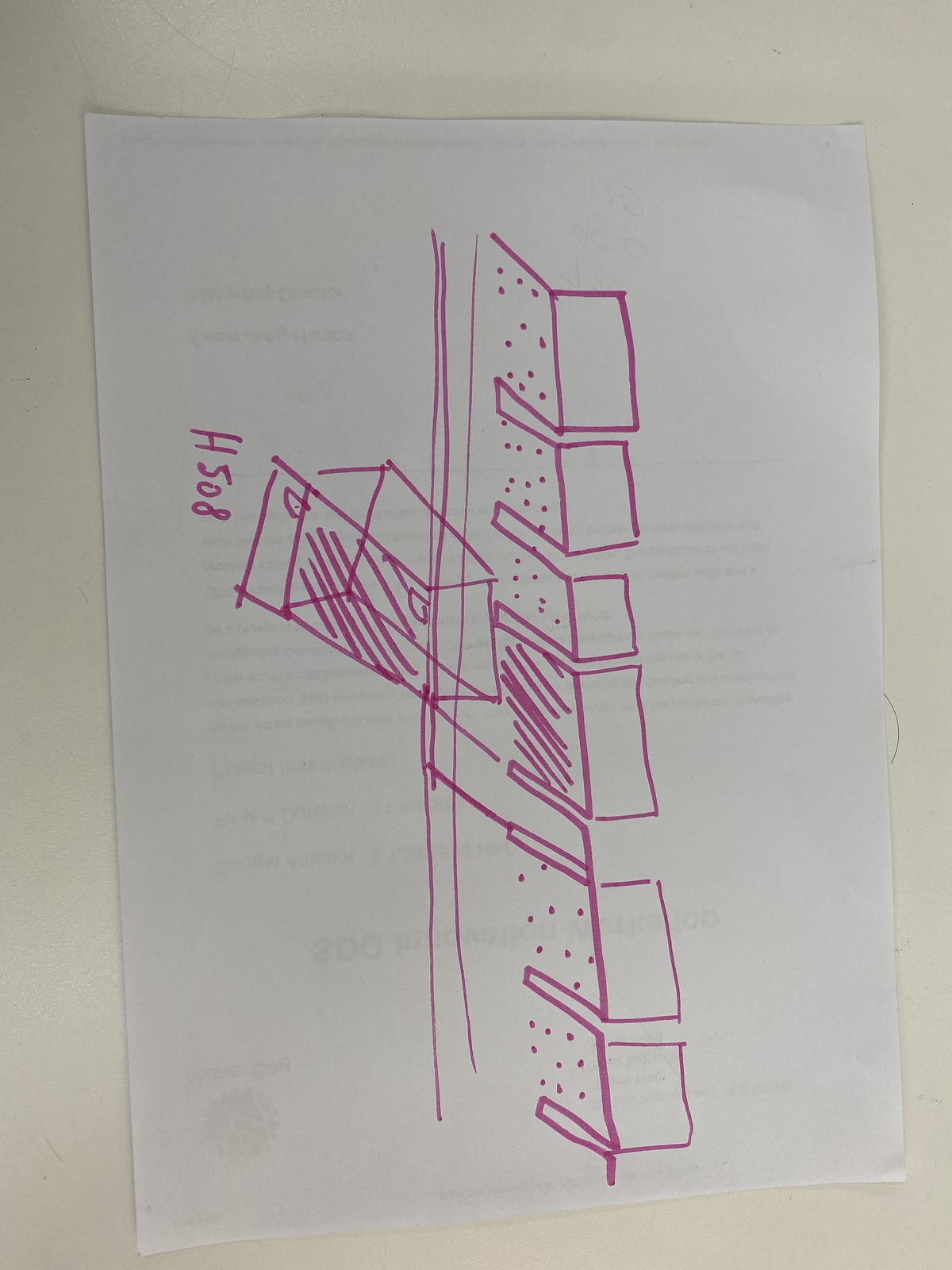A white sheet of paper, flipped so that only its blank side is visible, serves as the canvas for an intriguing, vertical hand-drawn sketch. In the top left corner, "H508" is scrawled in pink marker. The sketch predominantly features a series of shapes resembling various rectangles and possible teeth marks, aligned in a manner that evokes the layout of piano keys or perhaps a type of brush or curb.

The primary area of the drawing includes a 3D-rendered box with hash marks, which gives the illusion of a rectangle with a transparent top and hashed bottom. Attached to this box are three nearly vertical lines, extending nearly the entire length of the paper. In front of these lines are smaller, incomplete 3D rectangles—each lacking a defined bottom edge.

Each of these rectangles has variously placed purple dots lining the top edges. The pattern of dots continues through the initial three rectangles. The fourth rectangle then differs, featuring hash marks on the top. Following this, two more incomplete rectangles appear at the bottom, lined with additional dots. The sketch suggests a continuation of this pattern, but the paper runs out of space, leaving the drawing unfinished.